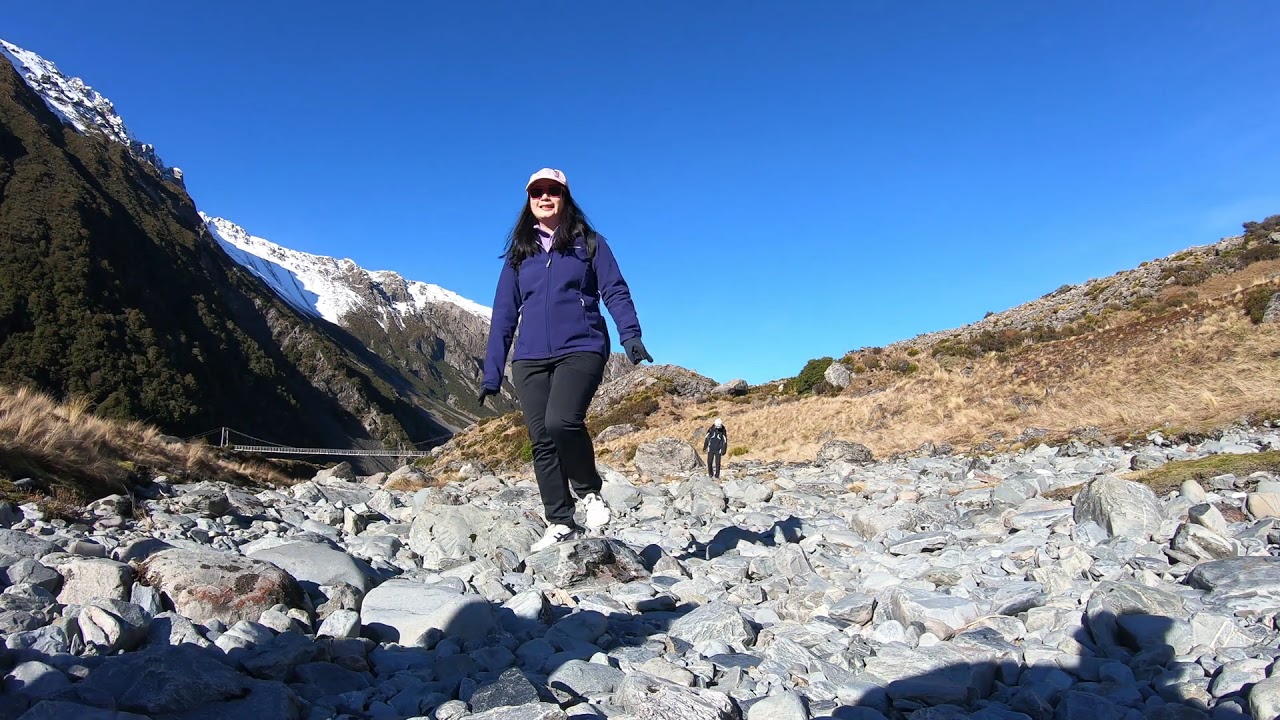In this horizontally aligned rectangular image, a clear blue sky with no clouds stretches across the top, above majestic, snow-capped mountains. The left side of the mountains features dark brown peaks dusted with snow, while a shorter, light brown hill dominates the right side. Nestled amid the mountainous terrain, a bridge spans an indentation between the peaks.

In the foreground, a rocky terrain of large gray rocks covers the lower part of the image. At the center, a woman walks towards the camera, clad in black pants, white shoes, and a long-sleeved navy jacket. She sports a white baseball cap and sunglasses, her long, dark hair cascading down. On her left, the imposing, snow-touched mountains rise, adding to the grandeur of the scene. Far behind her, another person dressed in dark clothing can be seen walking on the rocks, their figure too distant to reveal specific details. The combined elements of rocks, mountains, and human figures create a striking outdoor setting that captures both the beauty and challenge of the rugged landscape.